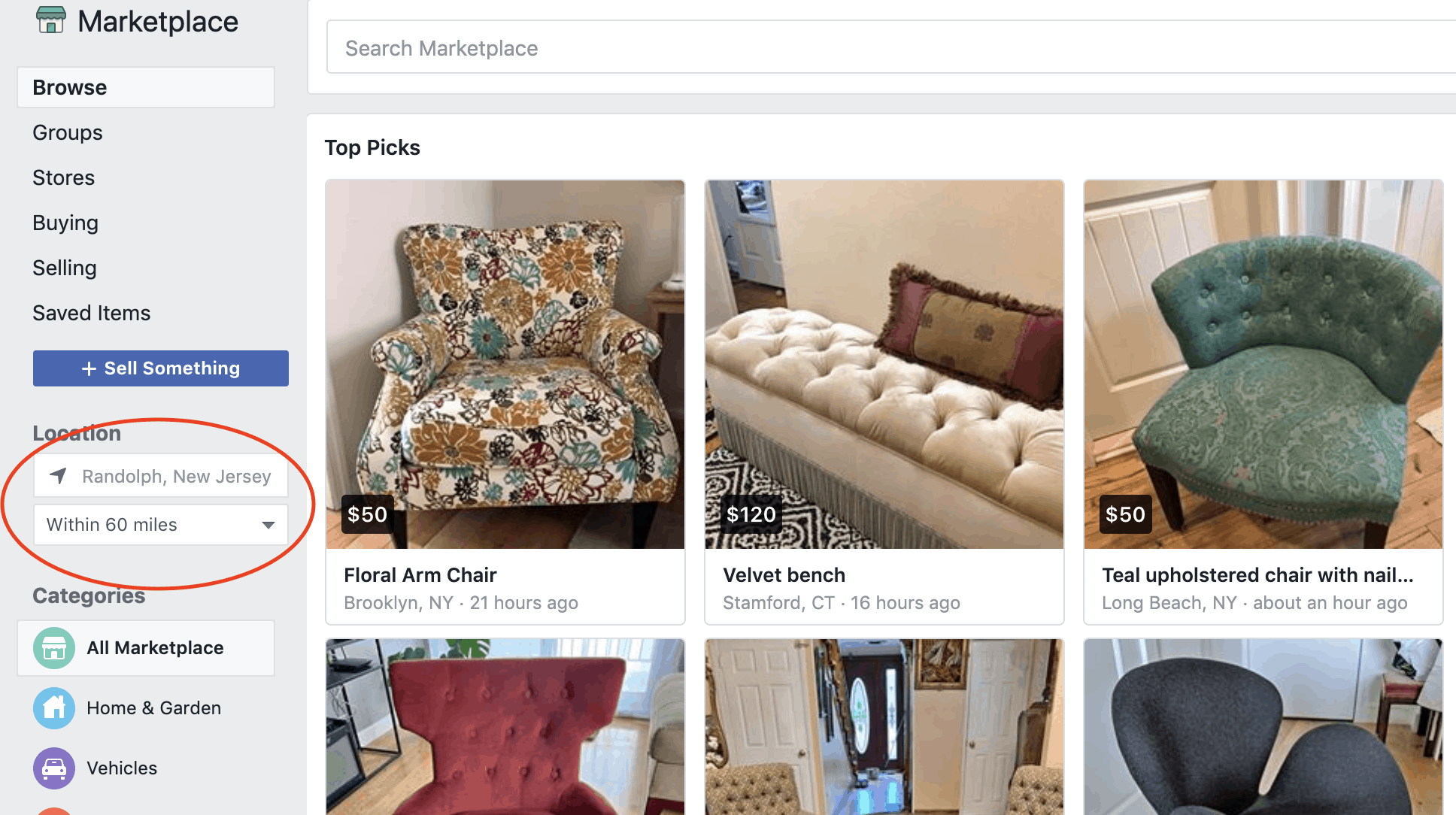The image depicts an online marketplace interface, prominently labeled "Marketplace" in the upper left corner accompanied by a house icon. At the top of the interface, there is a search box labeled "Search Marketplace." Below this, a left-hand column displays several navigation options: Marketplace, Browse, Groups, Stores, Buying, Selling, and Saved Items. A large blue rectangular button labeled "Sell Something" is also present in this column.

The user has set their search parameters to within 60 miles of Randolph, New Jersey, specifically focusing on furniture. The listings showcase six used furniture items. The first listing is a floral armchair priced at $50, followed by a velvet bench available for $120. Next is a teal upholstered chair with nailhead trim, priced at $50. Additionally, there are three more chairs partially visible in the images, but their descriptions are lacking, showing only the backs of the chairs. Notably, there is a red oval marking around the location section for emphasis.